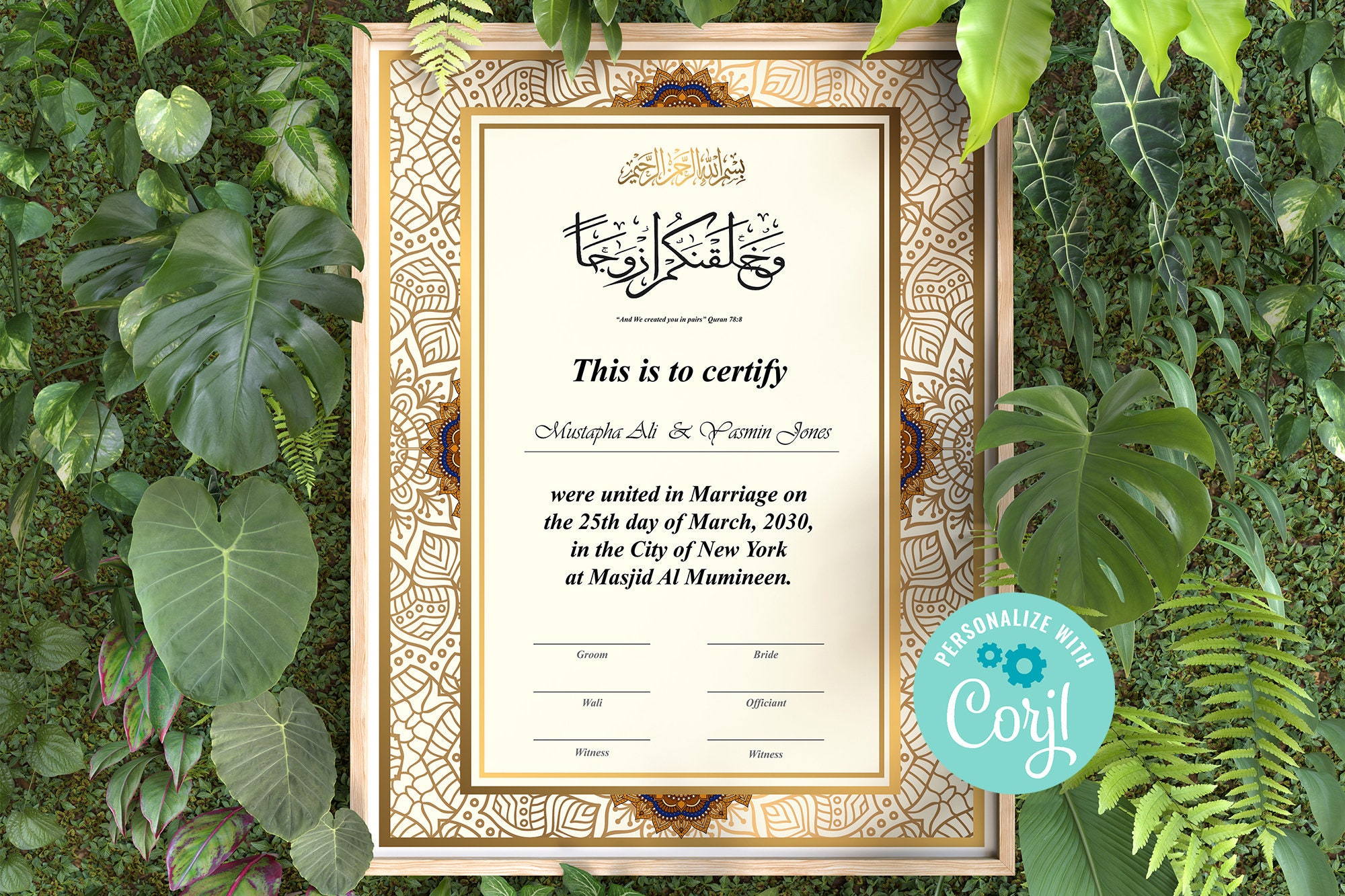A beautifully designed marriage certification document with a bronzy wooden border accented by an intricate brown and white design. The certificate gracefullly states: "This is to certify that Mustafa Ali and Pasmine Jones were united in marriage on the 25th day of March 2030 in the city of New York at Masjid al-Mumineen." The background of the certificate is adorned with lush green ivy and foliage, adding a touch of nature's elegance. At the bottom, a small light blue and white circle bears the words "personalized with coral," showcasing the creator's personalized craftsmanship. This image appears to be an advertisement for bespoke marriage materials, highlighting the designer's attention to detail and artistic flair.